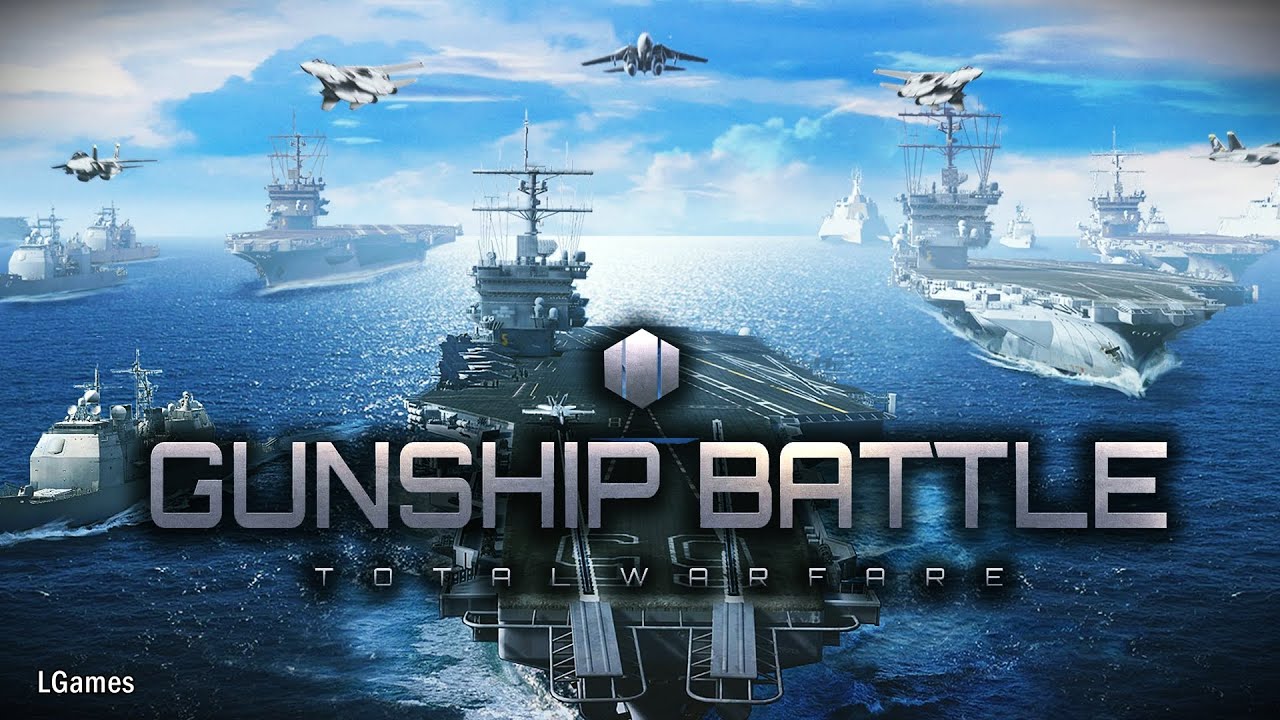This illustration, created for the video game "Gunship Battle: Total Warfare," prominently features a striking naval scene. The centerpiece is a large aircraft carrier at the forefront, surrounded by three additional carriers in the background. Several smaller gunboats and destroyers are also depicted, sailing in a formation that converges towards the viewer, suggesting an impending battle. The ocean is a deep, dark blue, while the sky overhead is a light blue with a scattering of clouds, hinting at a clear day. Above the naval fleet, five white fighter jets fly in a V formation, adding to the dynamic and intense atmosphere of the scene. The title "Gunship Battle: Total Warfare" is boldly superimposed over the central aircraft carrier, with a hexagonal icon divided into three sections positioned above the "P" in "Gunship." In the bottom left corner, the logo for L Games is visible, further anchoring the image as promotional material for the game.